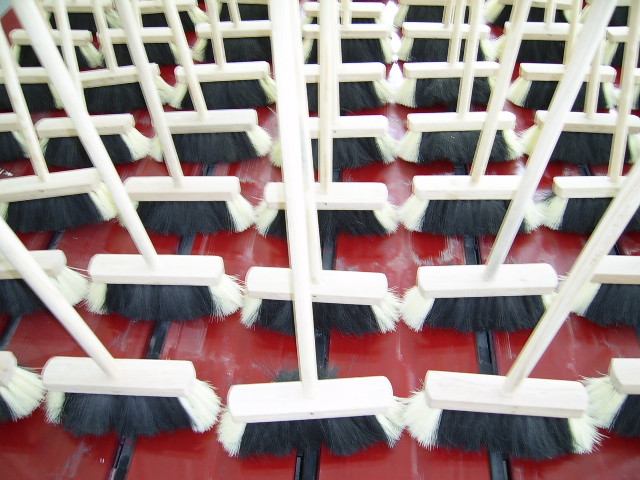This detailed photograph captures an impressive array of push brooms standing upright in a meticulously organized formation. The brooms, all identical, feature long white handles and rectangular bases where the bristles are attached. These bases are slightly curved on the ends and made of a plastic-like material. Each broom's bristles are predominantly black, with clusters of white bristles flanking both edges, creating a skunk-like appearance. 

The brooms are arranged in neat rows and columns, extending into the distance. The image appears to have been taken from a slightly elevated angle, offering a clear view of the bristles and the orderly alignment. The photograph is zoomed in enough that the tops of the handles are out of frame, yet the emphasis on the uniformity and the industrial, commercial-style design of the brooms is unmistakable.

They rest on a highly polished, red floor with thin black stripes running vertically between the red planks, suggesting a well-used, durable surface, possibly of wood or metal. The flooring appears slightly worn, with noticeable reflections and areas where the finish has faded or been scratched, hinting at the high-traffic nature of this setting. Overall, the image portrays an endless, almost hypnotic repetition of brooms, emphasizing their symmetry and the stark contrast of the red, black, and white color palette.